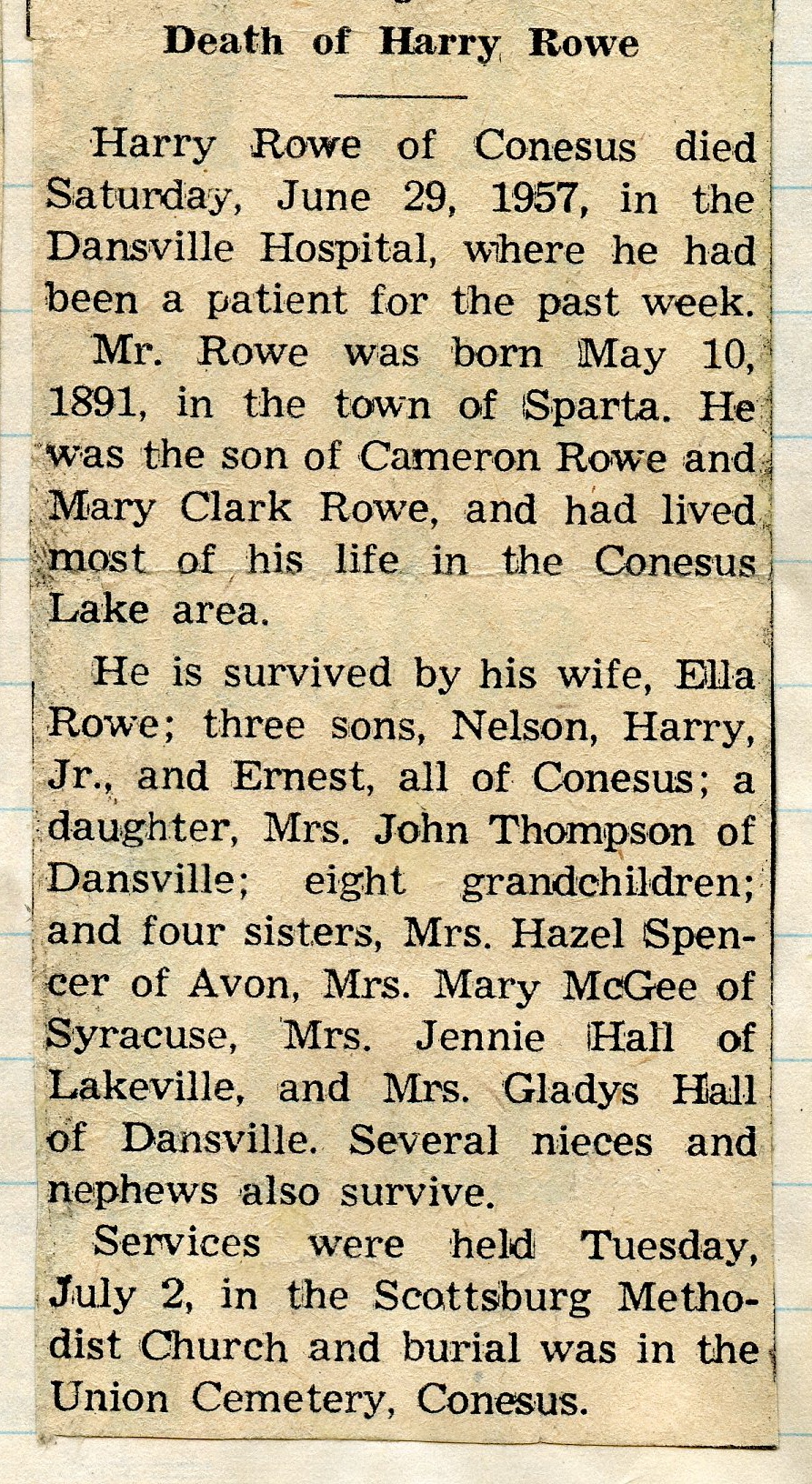The image is a photograph of an old yellowed newspaper obituary for Harry Rowe, pasted on a piece of school paper with blue horizontal lines. The obituary headline prominently reads "Death of Harry Rowe." According to the article, Harry Rowe of Conesus died on Saturday, June 29, 1957, at Dansville Hospital, where he had been a patient for the past week. Harry Rowe was born on May 10, 1891, in Sparta, the son of Cameron Rowe and Mary Clark Rowe. He spent most of his life in the Conesus Lake area. He is survived by his wife, Ella Rowe; three sons, Nelson, Harry Jr., and Ernest, all of Conesus; a daughter, Mrs. John Thompson of Dansville; eight grandchildren; and four sisters, Mrs. Hazel Spencer of Avon, Mrs. Mary McGee of Syracuse, Mrs. Jenny Hall of Lakeville, and Mrs. Gladys Hall of Dansville. Several nieces and nephews also survive. The services were held on Tuesday, July 2, at the Scottsburg Methodist Church, with burial in the Union Cemetery in Conesus.